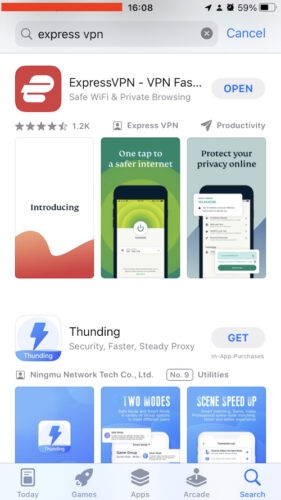This image is a screenshot captured from an iPhone, showcasing the Apple App Store interface. The background is predominantly light, with a distinctive silver header at the top that includes a search bar. The user has input the term "ExpressVPN," clearly visible in the search field.

Directly below, the listing for ExpressVPN appears prominently. The app’s recognizable logo, an abstract red design incorporating an "E," is displayed alongside its name, "ExpressVPN - VPN for WiFi & Private Browsing." To the right of the app name, an "Open" button is visible, indicating that the application is already installed on the device.

Underneath the ExpressVPN listing, there are three promotional thumbnails highlighting its key features. The images serve as a visual advertisement, detailing what users can expect from the app.

Below the ExpressVPN listing is another app named "Thunding." Its icon features a striking blue lightning bolt. Unlike ExpressVPN, the "Get" button to the right of Thunding’s name suggests that this app is not currently installed on the device. Additionally, this listing includes three blue-themed images, presumably illustrating the app's functionality and user interface.